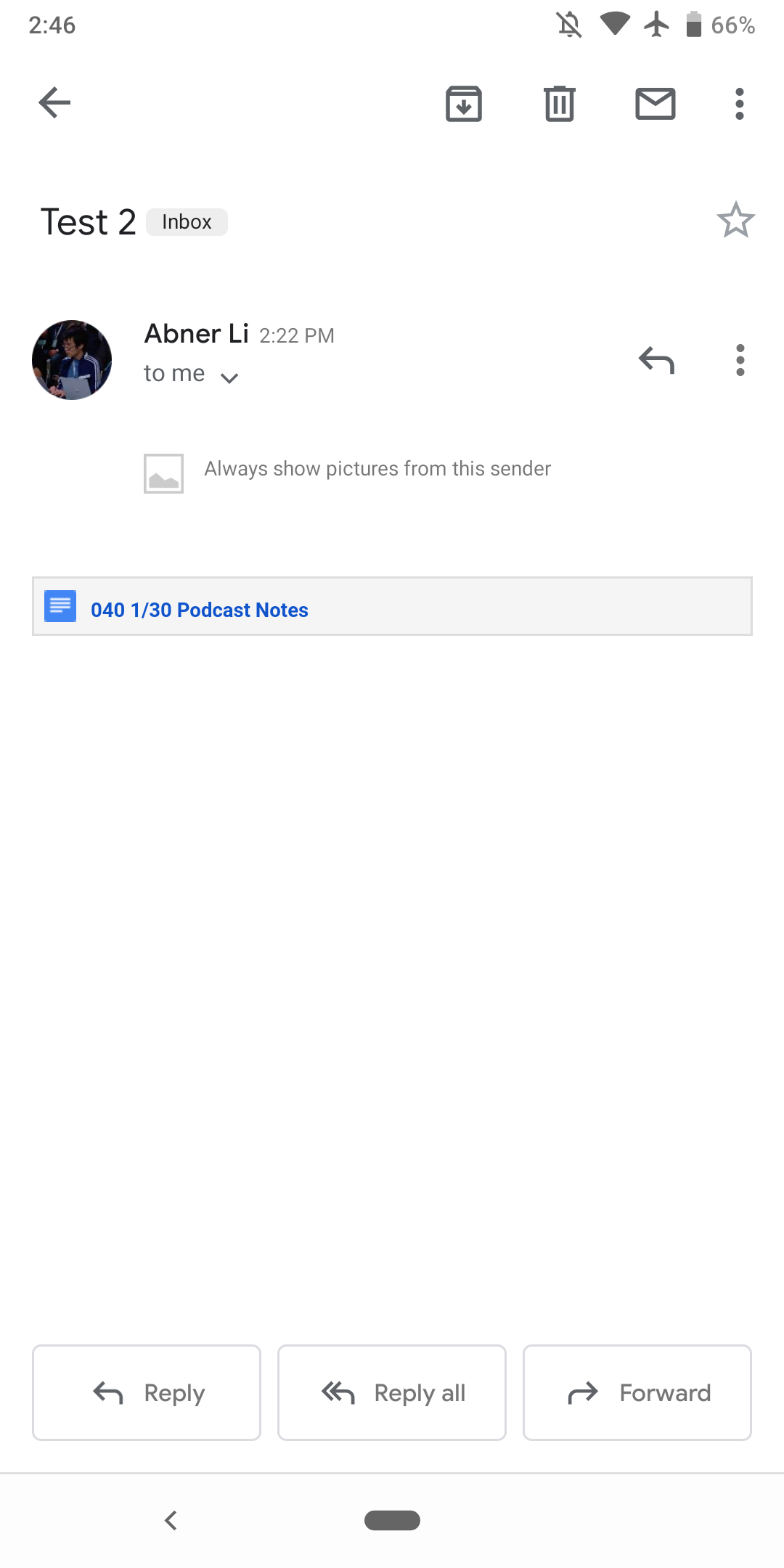The image depicts a mobile interface design set against a minimalist white background. 

- **Top Left:** The current time is displayed as "2:46" in gray text.
- **Top Right:** Icons for notifications (crossed out), full Wi-Fi signal, airplane mode, and a battery icon showing "66%" battery life.
  
- **Function Icons:** Below the status bar, there are four icons arranged horizontally:
  - A leftward-pointing back arrow.
  - A download icon.
  - A trash bin icon.
  - A compose message icon.

- **Email Interface:**
  - The title "Test 2" is displayed above an inbox label, accompanied by a star icon to mark the email as a favorite.
  - A profile image of a man with brown hair wearing a blue and white tracksuit is shown next to the sender's details.
  - Text description: "Interlay Abner Li, 2:22 PM, to me. Always show pictures from this sender."
  - The email subject reads: "040 one of 30 podcasts notes," which could also be interpreted as "1 of 30's podcast notes."

- **Action Buttons:** At the bottom of the screen, there are options to "Reply," "Reply All," and "Forward."